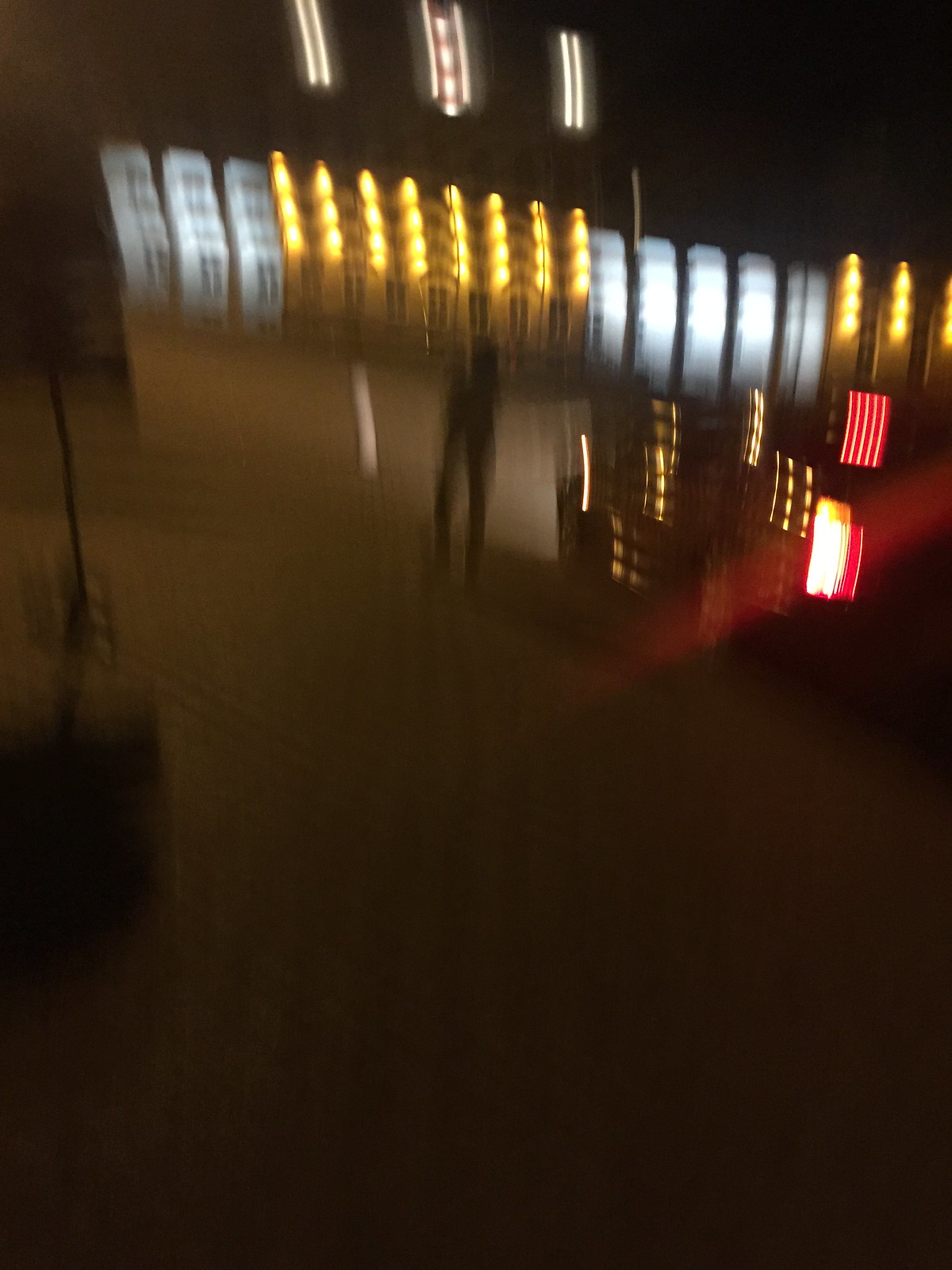A blurred photograph captures a nighttime street scene with a vehicle, likely a car, discernible by its faintly visible two wheels and rear lights. The image also includes a dark figure standing on a gray or brown sidewalk. In the background, there's a building adorned with illuminated windows or doors, featuring vertical rows of yellow lights in the center, flanked by tall, bright white lights on both sides. A street sign is also faintly visible within the frame, adding to the urban ambiance of the scene.